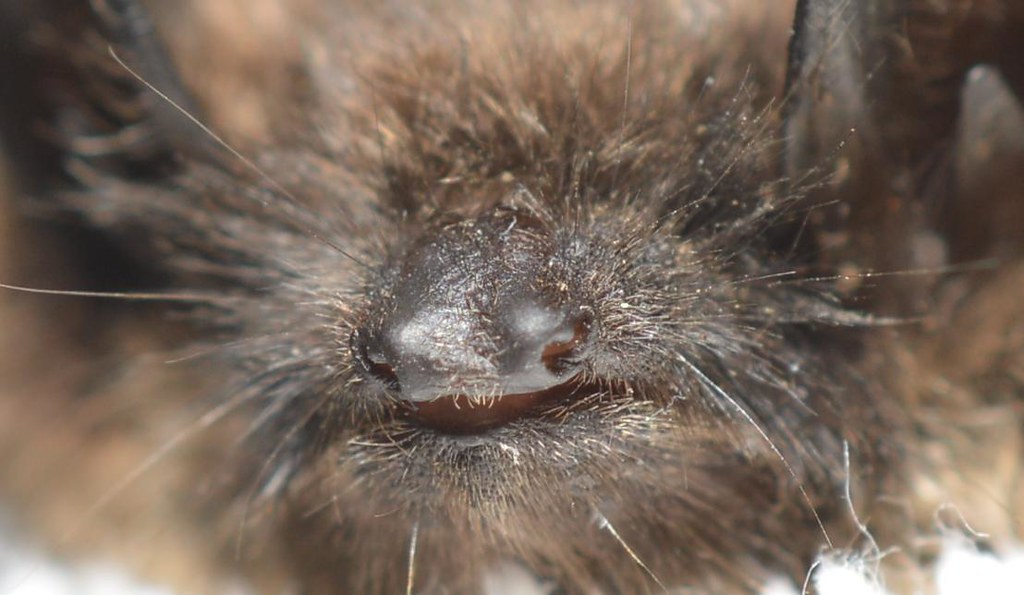In this highly detailed close-up image, we see a creature with a striking and somewhat menacing appearance. Its face is predominantly black, contrasted by a chaotic mane of fur that ranges from brown to black, giving it a wild and untamed look. The creature, which could be mistaken for a little fish at first glance, has an intense, almost intimidating presence, accentuated by its strange, beady black eyes. The dense fur enveloping its body adds to its eerie and mysterious appeal, leaving viewers uncertain if they're looking at an unusual fish or a possibly a large, furry spider.